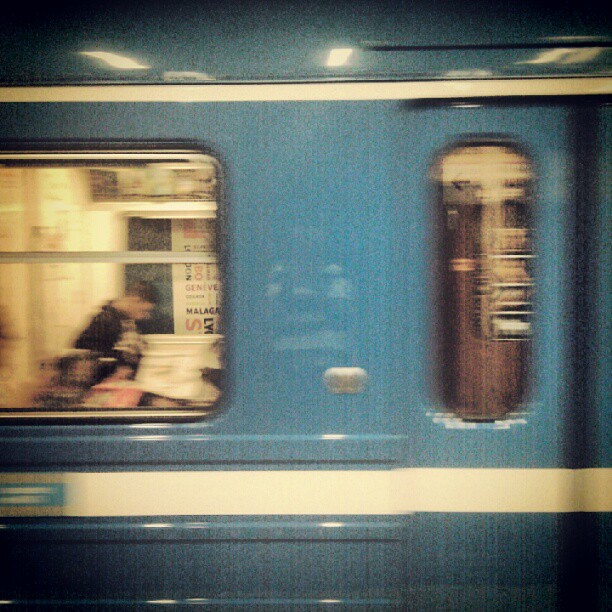The image captures a moving blue train, its blurred motion conveying a sense of speed. Along its length, you can see distinct horizontal white lines, one near the bottom and a smaller one near the top. Prominently visible through a large window on the left side of the train, a gentleman with short hair, dressed in a black shirt, seems engrossed in reading something, likely a newspaper. Adjacent to this window, a smaller oval window, perhaps part of a door, offers another point of view. Inside, behind the gentleman, there's a partially obscured poster with red, black, and orange letters, difficult to make out due to the image's graininess. Additionally, on the bottom left white stripe of the train, a small blue placard with indistinct white writing adds another layer of detail to the scene.